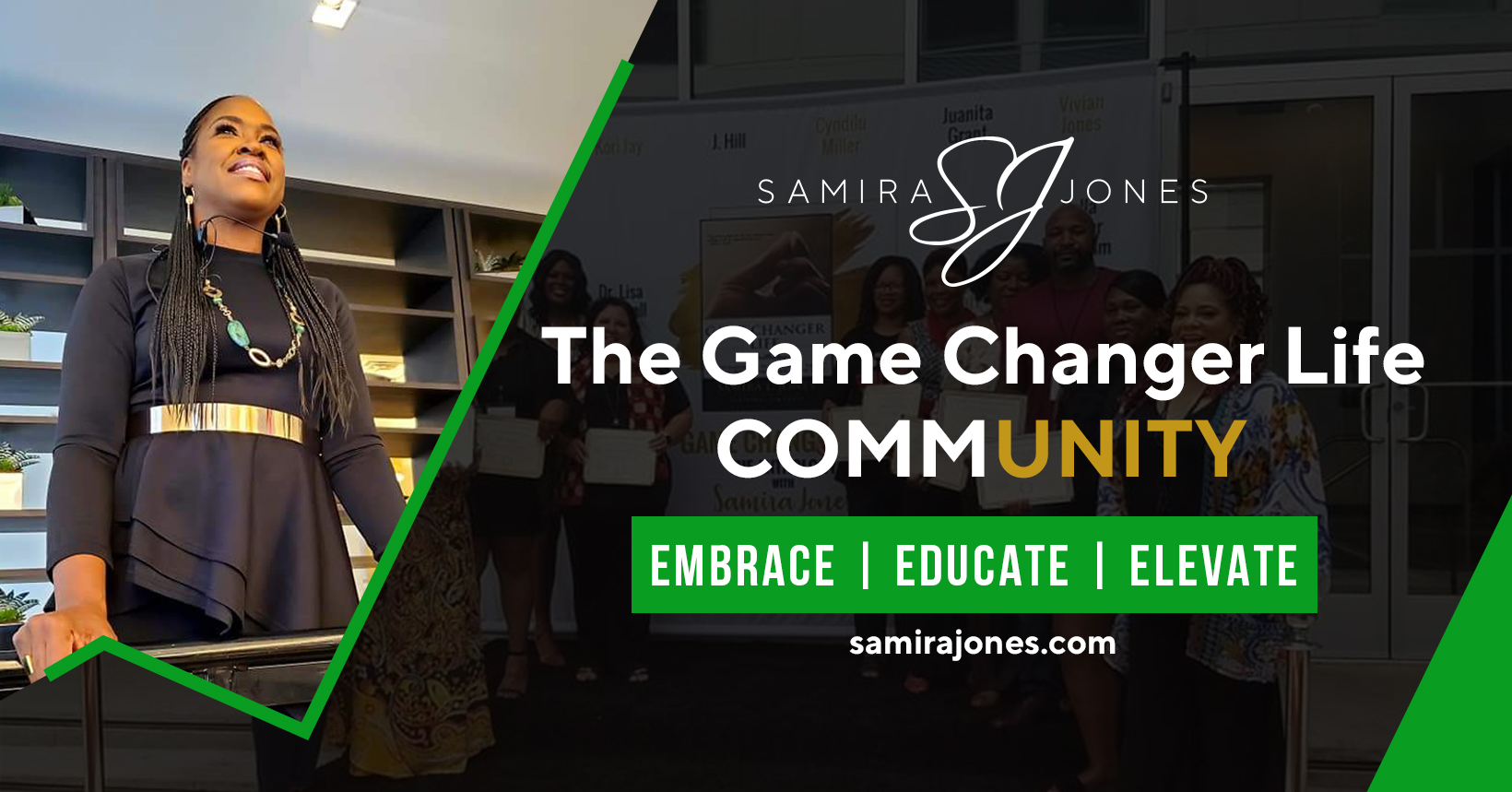This horizontal advertisement features Samira Jones, a black woman with long dreadlocks, depicted facing what appears to be a group of people. She is well-dressed in a long-sleeved, flowy black T-shirt with a gold stripe across the middle, which also resembles a belt, and she accessorizes with a large necklace. Samira is smiling warmly, likely addressing her audience, set against black shelves whose contents are unclear. To the right, the advertisement features a dark background with a black filter and emphasizes text in white that reads "Samira Jones, The Game Changer Life Community." Below this, in a green-outlined rectangle with white text, are the words "EMBRACE, EDUCATE, ELEVATE." A green triangle is located in the lower right corner of the image, and her website, samirajones.com, is prominently displayed. The background incorporates elements of black, green, and white, contributing to the professional and motivational tone of the advertisement.